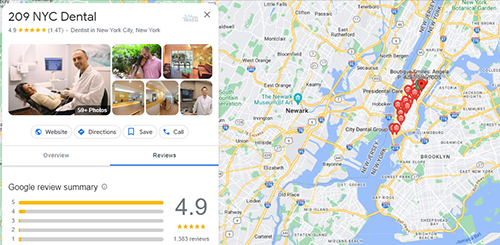Here's a detailed and cleaned-up caption for the given image description:

---

**Image Caption:**

The image features a smaller advertisement for "209 NYC Dental" on the left side of the screen. The top of the ad prominently displays the clinic's name in white text against a black background. To the right of the name, there's a close button (a grey "X" mark). The clinic boasts a rating of 3.9 stars. The snippet includes the location as New York City, NY.

In the main focus of the image, a smiling woman is seated in a dentist's chair, while a dentist stands beside her, both looking directly at the camera. The woman's smile appears overly enthusiastic, while the dentist exhibits a more reserved expression, as if surprised by the photo being taken.

Surrounding this main photo are additional images showcasing different areas of the dental office, offering a glimpse into the clinic's environment.

Below the images, there are several clickable options such as "Website," "Directions," "Save," "Call," "Overview," and "Reviews." Additionally, there's a summary indicating the clinic's Google reviews: a high rating of 4.9 out of 5 stars from a total of 1,383 reviews, which includes a mix of ratings (including five-star, four-star, three-star, two-star, and a noticeable number of one-star reviews).

The image also includes a pulled-back view of a Google Map highlighting the location of the clinic in New York City. The map shows surrounding areas like Newark, New Jersey, Brooklyn, and Manhattan. Multiple red dots with small white house icons are scattered across Manhattan, suggesting the business has several locations in the area.

---